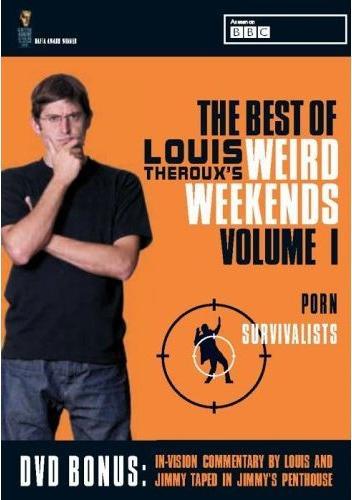This is a photograph of a DVD cover titled "The Best of Louis Theroux's Weird Weekends Volume 1." The cover features an orange background with two black borders at the top and bottom. Prominently placed on the left side of the cover is Louis Theroux, depicted with short brown hair, glasses, a black T-shirt, and blue jeans. In a pensive pose, he holds his chin as if deep in thought. The title text is in bold black lettering, except for "Weird Weekends," which is in white. Above the title, there's a "As Seen on BBC" label on the top right corner. To the right of Louis is a person in a target marker, consisting of a silhouette enclosed within concentric circles and dashed lines, indicating a focus point. The bottom of the cover highlights a special feature, stating "DVD Bonus: Envisioned Commentary by Louis and Jimmy taped in Jimmy's penthouse." The DVD focuses on the unique category of "Porn Survivalists."